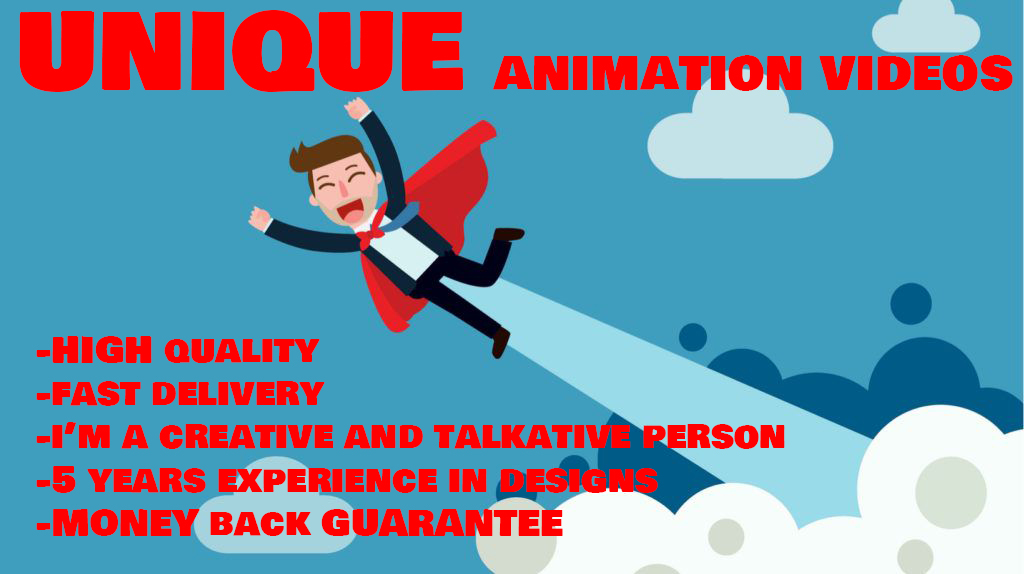This cartoonish advertisement banner, reminiscent of online ads, features a prominent headline at the top in bold red text that reads "Unique Animation Videos." Set against a cerulean blue background, the central image depicts a man with brown hair, a joyful expression, and a red cape, dressed in a business suit with a blue tie. He appears to be flying like Superman from the bottom right to the top left, leaving behind a light blue trail. Surrounding him are various clouds ranging from off-white to dark blue. Along the left edge, in red lettering, there are five key points listed: "High Quality," "Fast Delivery," "I'm a Creative and Talkative Person," "Five Years Experience in Design," and "Money Back Guarantee."